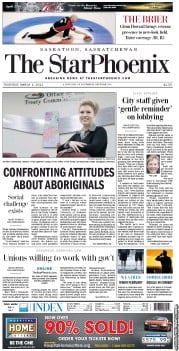Front Page of The StarPhoenix Newspaper

This is a detailed depiction of an almost nostalgic sight—the front page of a newspaper. The newspaper is identified as "The StarPhoenix," prominently displayed in large letters a little way down the page beneath an advertisement. Although the image is slightly out of focus, some key elements are discernible. 

At the center of the page, there is a photograph of a woman positioned on the right side. She is dressed in a buttoned-up shirt worn underneath a black long sleeve shirt. Her hair is pulled back, and her arms are crossed on top of the back of a chair. She appears to be Caucasian with white skin. The accompanying headline reads "Confronting Attitudes About Aboriginals."

To the right of this central image is a vertical column with the title "City Staff Given Gentle Reminder on Lobbying." The page's layout features two vertical portions of text on either side, which further split into sections. Embedded in the right column is another photograph, this time of a white female with short hair.

Both the top and bottom of the page include advertisements, framing the main content and signifying the commercial aspect of traditional print media.